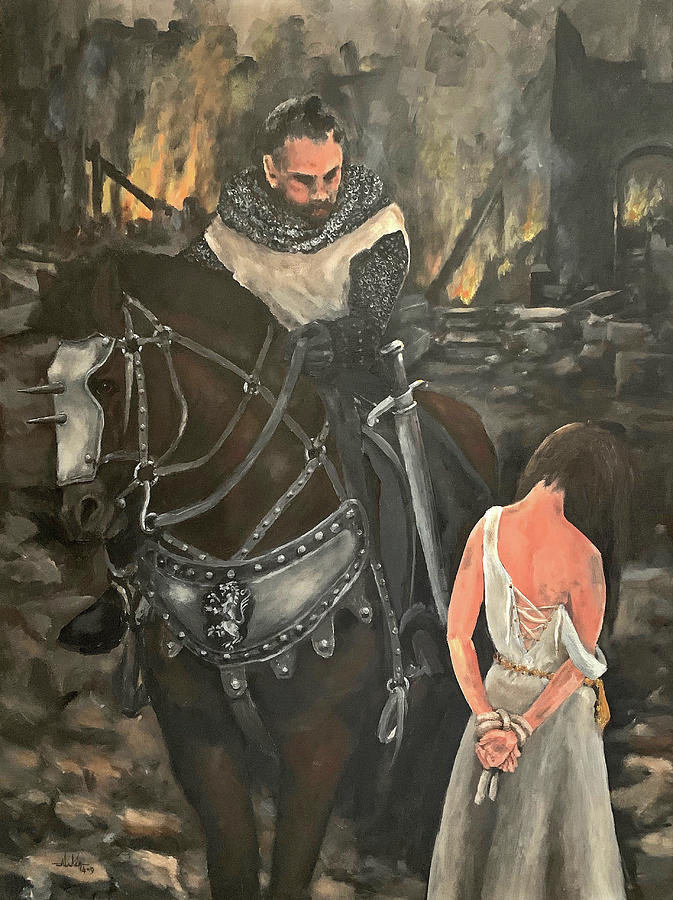A painted artwork with semi-realistic detail portrays a dark and ominous medieval scene. At the center, a white-skinned knight clad in chainmail armor and a white tunic, resembling a mix of Robin Hood and traditional medieval knights, sits atop a brown horse equipped with metal armor, heavy reins, and a front plate emblazoned with an emblem. The knight, whose expression is obscured, has a sword strapped to his saddle. Beneath him, to the fore and left, stands a woman with long brown hair cascading forward, her head hung low in shame. Her fair skin is marred with dirt, and her hands are tied tightly behind her back. Her tattered dress hangs loosely from one shoulder, suggesting recent violence. The background is filled with the ruins of a burning village, indicating the aftermath of a destructive conflict.